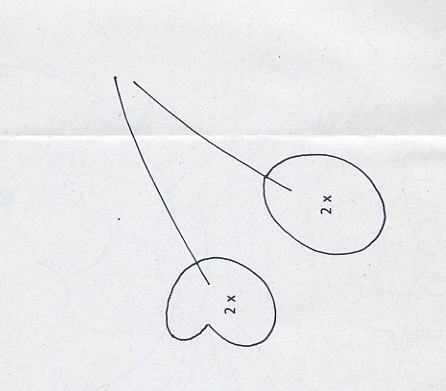A close-up image depicts a white sheet of paper folded horizontally, dividing the top third from the bottom two-thirds by a single crease. On the paper is a rudimentary drawing of two cherries with stems. The illustration consists of two lines and two shapes. The stems start near the top left corner, but not precisely at the edge, and diverge in a manner that resembles an inverted "V." One stem angles downward towards the middle-right side of the paper, while the other extends more vertically towards the bottom. The shapes at the ends of these lines are somewhat circular, with one leaning towards a heart-like form on the left and the other being more rounded on the right. Both shapes feature the characters "2 x" printed inside, separated by a space. The simplicity of the drawing is emphasized by the basic use of lines and forms, giving it a charming, almost childlike quality.